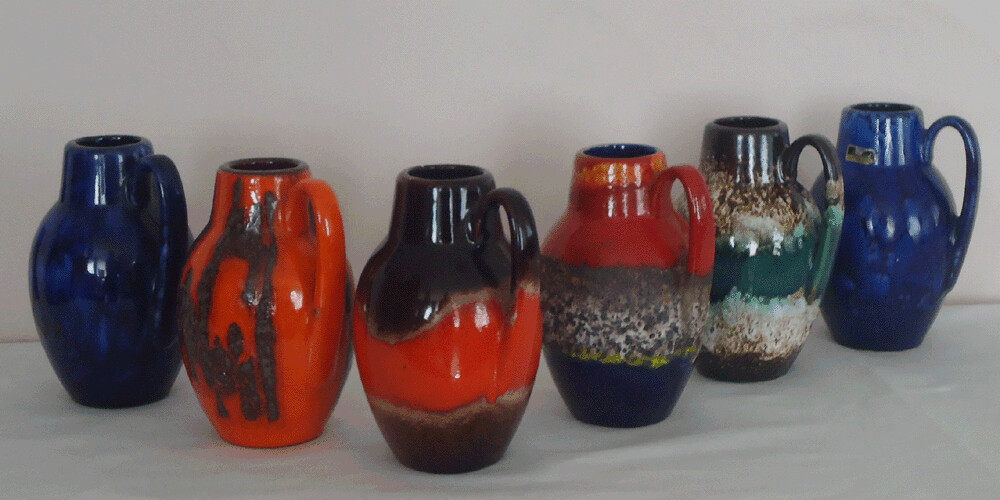This is a detailed picture of six intricately designed clay jug vases, arranged in a semi-circle atop a table draped with a white linen cloth, set against a stark white background. These jug vases, with their distinctive handles, are highly glazed and exhibit a brilliant, shiny finish suggestive of Greek artistry. Their colors are bold and varied: the one on the far left is a deep blue with lighter blue highlights illuminated by light; next to it, a burnt orange jug displays tribal-like brown markings. The third vase is predominantly dark brown with a striking wave of orange and gold in the center. The fourth jug combines shades of browns with touches of blue in a mottled pattern. A jade green vase follows, interspersed with mottled brown and cream hues. The final jug is a stunning deep blue, completing the vibrant array. Each piece is crafted with clay and fired in a kiln to achieve their high-gloss finish.